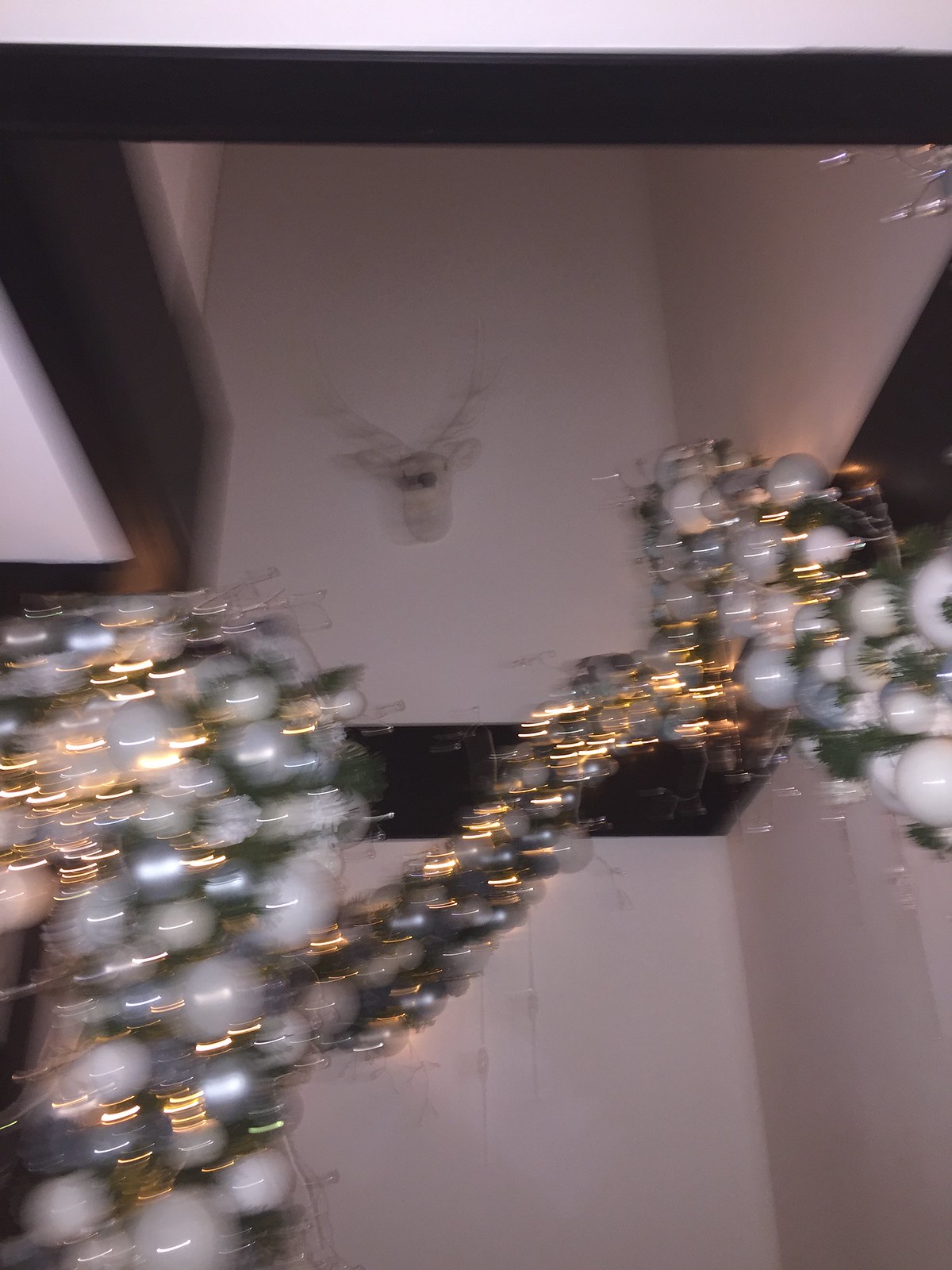In this out-of-focus photograph, a festive scene of Christmas decorations is captured within a stairwell. High above, nestled in the corner, hangs a charming white reindeer mask adorned with two round black eyes and petite antlers. The decorations feature a beautiful arrangement of white and silver Christmas balls intertwined with a lush green tinsel garland. Adding to the festive ambiance, radiant gold lights illuminate the display. The garland artfully ascends along the right side of the wall before elegantly draping down and connecting to a corresponding piece on the left side. Separating the first floor from the second is a dark wood border, adding a touch of classic elegance to the holiday display.